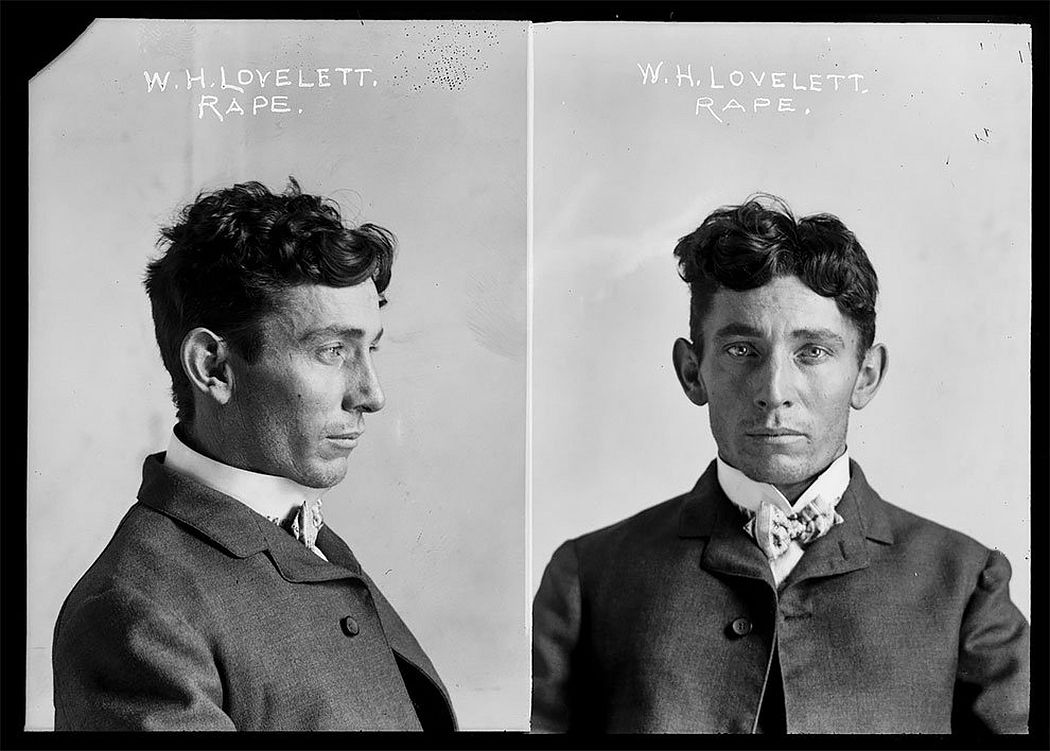This image features an old black and white mugshot from what appears to be the early stages of photography, likely the early 1900s. The compilation consists of two photographs of a young man, possibly in his 30s, set indoors with a gray background and enclosed within a black border. Both images display the man identified as "W.H. Lovett" with the word "Rape" written above each photo in white letters.

The left photograph shows the man in profile, facing left. He is wearing a black 19th-century style suit with a white collared shirt and a bow tie. In this profile view, his short, curly hair is prominently displayed, particularly around his ears. On the right, the same man looks directly at the camera with a somber expression; his short curly hair, clean-shaven face, and large ears are clearly visible. His eyes appear open and alert, though their color is indistinguishable due to the black-and-white medium. The overall style and appearance of the photograph and attire suggest it is not contemporary but rather a historical document.